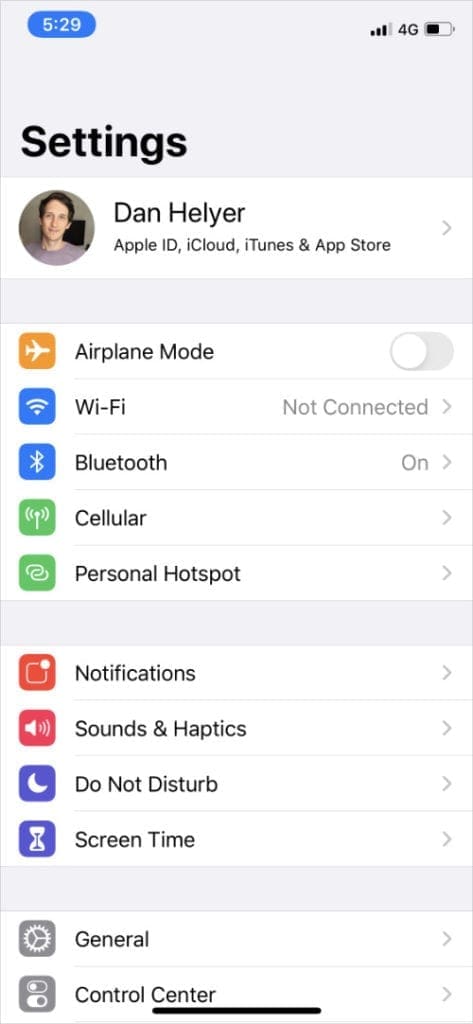This image depicts the Settings screen of an iPhone. In the upper left corner, the time is displayed within a blue bubble, showing 5:29 in white numerals. To the right, the cell signal strength, the 4G connectivity indicator, and the battery icon are visible. 

Prominently centered, the word "Settings" is written in bold black letters. Below this, the name "Dan Helyer" is displayed, indicating the Apple ID of the user. This section also provides access to the user's iCloud, iTunes, and Apple Store accounts.

The screen lists various setting options starting with "Airplane Mode," which is currently turned off. Following this, "Wi-Fi" is shown as not connected, while "Bluetooth" is enabled. The "Cellular" and "Personal Hotspot" sections are accessible but details are not provided in the image. Additional options include "Notifications," "Sounds & Haptics," "Do Not Disturb," "Screen Time," "General," and "Control Center." 

This image provides a comprehensive view of the primary settings available on the user's iPhone.